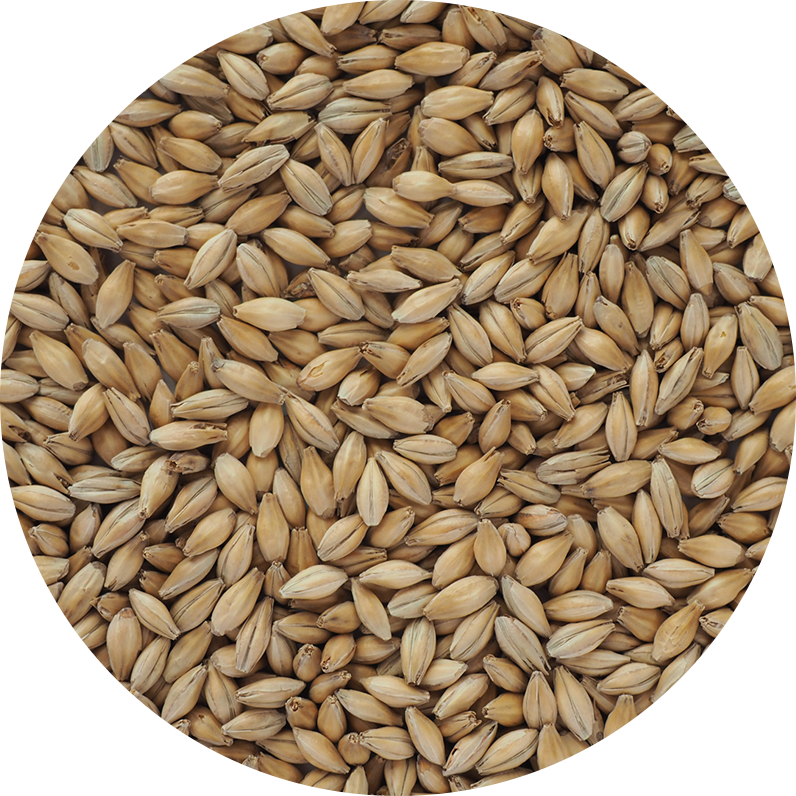The image is a close-up, overhead photograph of an array of beige, seed-like objects clustered together. Cropped into a perfectly round shape with a white background, the depiction shows these seed-like structures—resembling elongated pistachios still in their shells—arranged haphazardly, with most positioned side-to-side and some oriented up-and-down. Despite their varied directions, their coloration ranges from light cream to camel to light brown, and many exhibit a dark line running down the middle, indicative of where they might split open. The seeds fill the entire circular frame without any visible container, creating a visually engaging mosaic of natural textures and earthy tones.